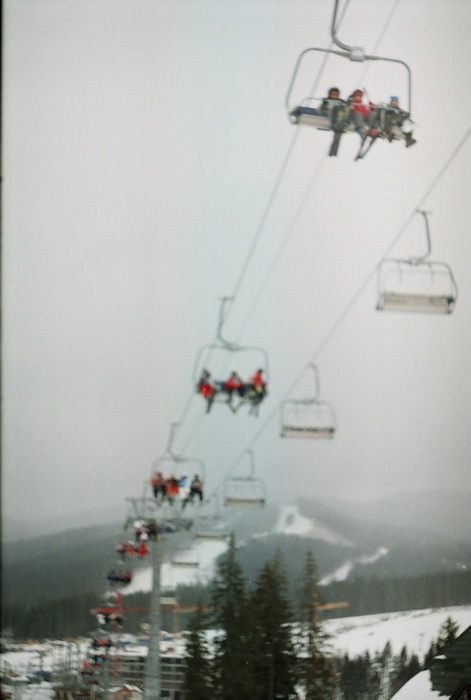In this vertical photograph of a ski resort, a grayish sky looms over a snowy mountain landscape with a ski lift stretching diagonally from the lower left to the upper right of the image. The ski lift, consisting of black cables connected to tall, gray metal poles, features open, rectangular seats where skiers sit, secured by a horizontal bar. On the upward track, each lift is filled with people, visible in varied attire: a prominent group in the upper right corner includes a person in a red outfit and two in gray, one with a blue hat. Another noticeable group in the midsection of the lift has individuals in red and black outfits. The downward track appears vacant. At the base of the image, a patchy cover of snow blankets the ground, dotted with evergreen trees, which become denser towards the middle and background, where the landscape ascends into snow-covered mountain peaks and continues under the uniform gray sky.